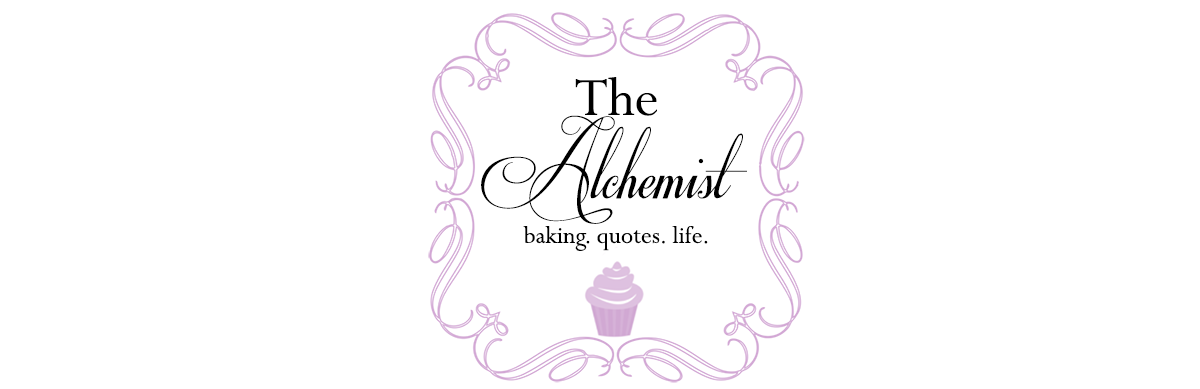This image features a meticulously designed PNG logo for a company or website. Encased by a scrolling border with elegant curly cues in a light purple-pink hue, the logo has a sophisticated yet playful aesthetic. The border forms a squared-off shape that surrounds the central elements of the design. 

Within this frame, the name "The Alchemist" is prominently displayed in an ornate, fancy scripted font. Below, the words "Baking. Quotes. Life." are aligned in smaller, simpler typography, each word separated by a period. 

At the bottom of the logo, a detailed computer graphic of a cupcake is prominently featured. The cupcake has inviting pink frosting with white accents, sitting in a slightly darker pink wrapper with noticeable folds, hinting at its realistic texture.

Measuring approximately 2 inches by 2 inches, the entire image rests on a translucent white background, maintaining a clean and professional look. The overall high-quality design suggests that this logo could effectively represent a brand on a website or in a newsletter, embodying both elegance and charm.